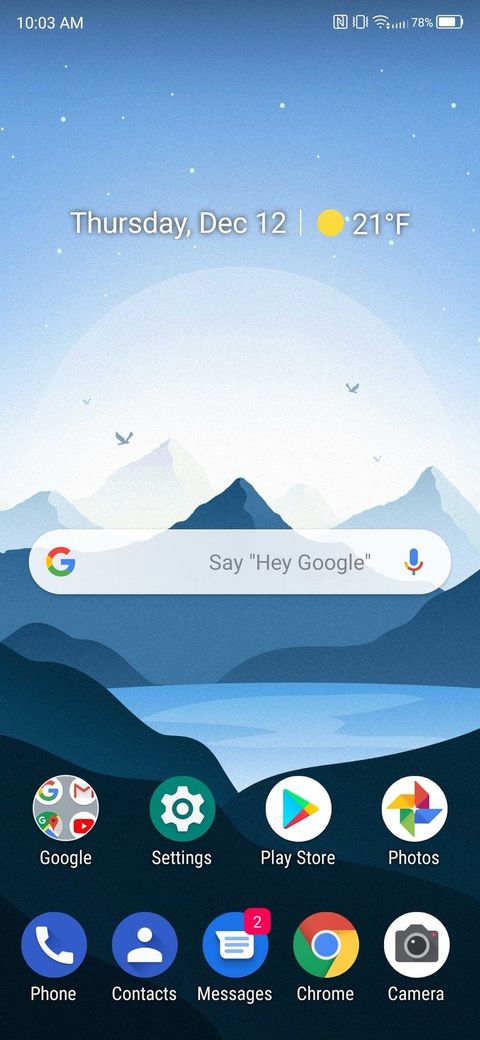This screenshot captures the detailed layout of a smartphone's homepage at 10:03 AM. The status bar at the top indicates that the phone is set to vibrate mode, the Wi-Fi signal is strong, and the battery is at 78%. The temperature is displayed as 21°F. The vibrant wallpaper depicts a serene scene with birds flying over mountains and a lake, complemented by the sun casting a bright glow. The background features various shades of blue with some white, and subtle stars dotting the upper portion of the screen. 

The date, Thursday, December 12th, is also displayed prominently. Just over halfway down the screen, there's a Google search bar enclosed in a capsule, complete with the "G" logo on the left and a microphone icon on the right. The phrase "Say hey Google" is shown in quotes within the search bar.

At the bottom of the homepage, there are two rows of app icons. The first row consists of grouped Google apps including Google, Gmail, YouTube, and Google Maps, alongside a settings app identified by a green icon with a gear symbol, the Play Store, and Photos. Below this, the second row includes icons for Phone, Contacts, Messages (which has an alert showing two new messages indicated by a red beacon in the upper right corner), Chrome, and Camera.